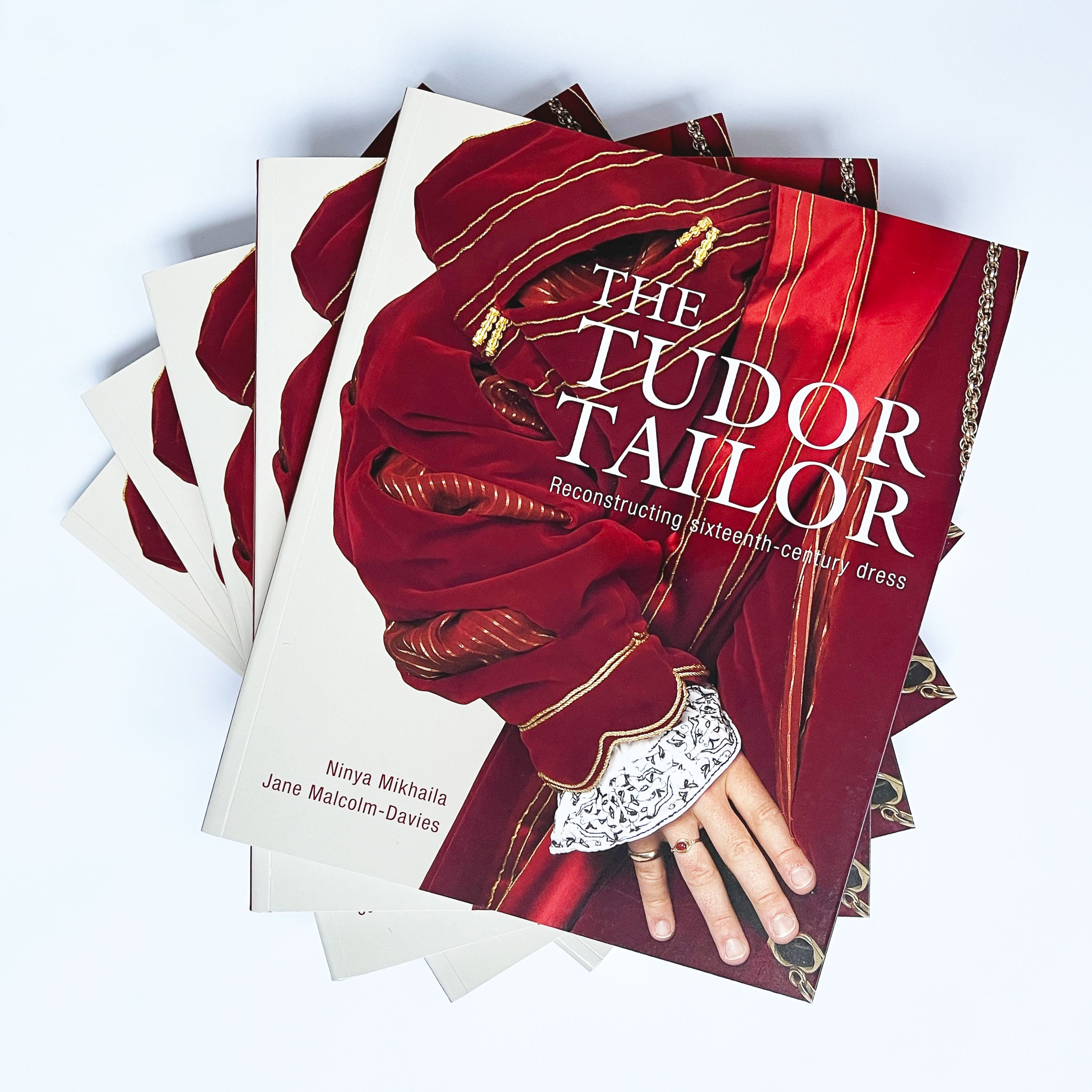This image features a neatly stacked set of five identical books, titled "The Tudor Tailor: Reconstructing 16th-Century Dress," authored by Nina Mikhaila and Jane Malcolm-Davies. The books are arranged in a staircase swivel pattern, allowing the corners of each book to be visible. The cover portrays a detailed illustration of a sleeve from a 16th-century robe—a dark red garment with gold stripes. The sleeve belongs to a figure adorned with rings on their fingers and a silver necklace, though only the arm, hand, and lower body down to just below the waist are shown. Set against a gradient background transitioning from blue to white, the image is framed by a plain white backdrop, drawing focus to the historical costume depicted on the book cover.